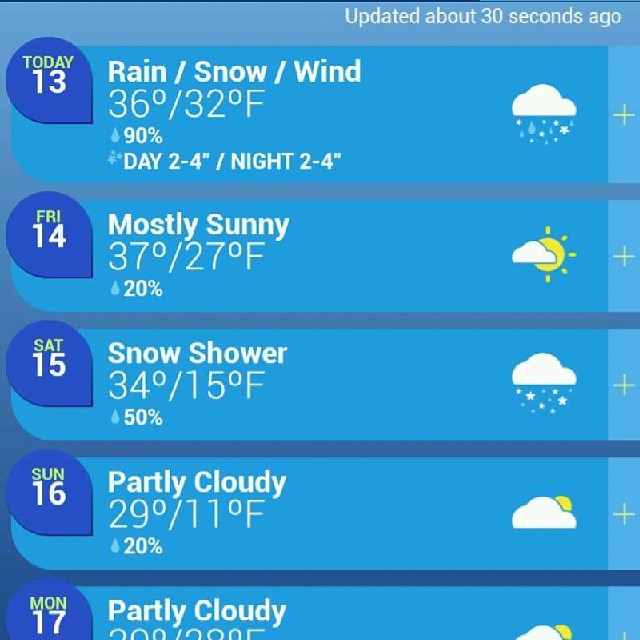The image is a screenshot of a weather app displaying a detailed forecast for the week. In the top right corner, it indicates it was last updated about 30 seconds ago. The forecast starts with today, the 13th, highlighting rain, snow, and wind, with temperatures ranging from 36 to 32 degrees Fahrenheit. There's a 90% chance of precipitation, with expected snowfall of 2 to 4 inches both during the day and night. For Friday, the 14th, it predicts mostly sunny weather with temperatures between 37 and 27 degrees Fahrenheit and a 20% chance of rain. Moving to Saturday, the 15th, snow showers are forecasted, with temperatures set at 34 and 15 degrees Fahrenheit, and a 50% chance of precipitation. Sunday, the 16th, is expected to be partly cloudy with temperatures of 29 degrees Fahrenheit and a 20% chance of precipitation. Next to each day's forecast, there are corresponding weather icons such as clouds with rain droplets and snowflakes for visual reference.